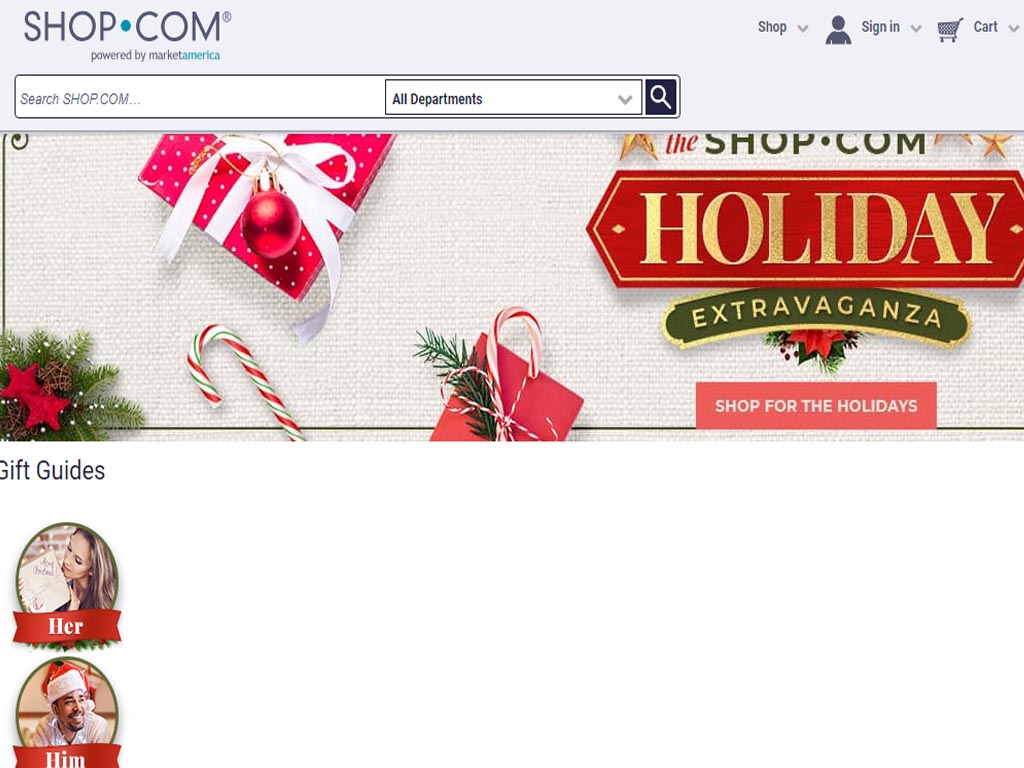This is a detailed screenshot of a shopping website, shop.com, which is powered by Market America. The website features a gray navigation bar at the top. On the left end of this bar, the shop.com logo is prominently displayed in gray text, with the dot and "America" in blue. Towards the right corner of the gray bar are three drop-down buttons labeled "Shop," "Sign In," and "Cart."

Beneath this header section is a search bar aligned to the left. The search bar has a text prompt that reads "searchshop.com," and includes a drop-down menu on its right side labeled "All Departments." Adjacent to the drop-down menu is a black, square-shaped search button.

Below the search bar, the site features a partially visible promotional banner for the shop.com holiday extravaganza. The right side of the banner showcases the text "shop.com holiday extravaganza." Here, "the" is in red, "shop.com" in green text, "holiday" in gold text framed by a golden border against a red background, and "extravaganza" in gold text within a green banner outlined in gold. Festive elements such as a red gift with a white bow are also displayed on the banner.